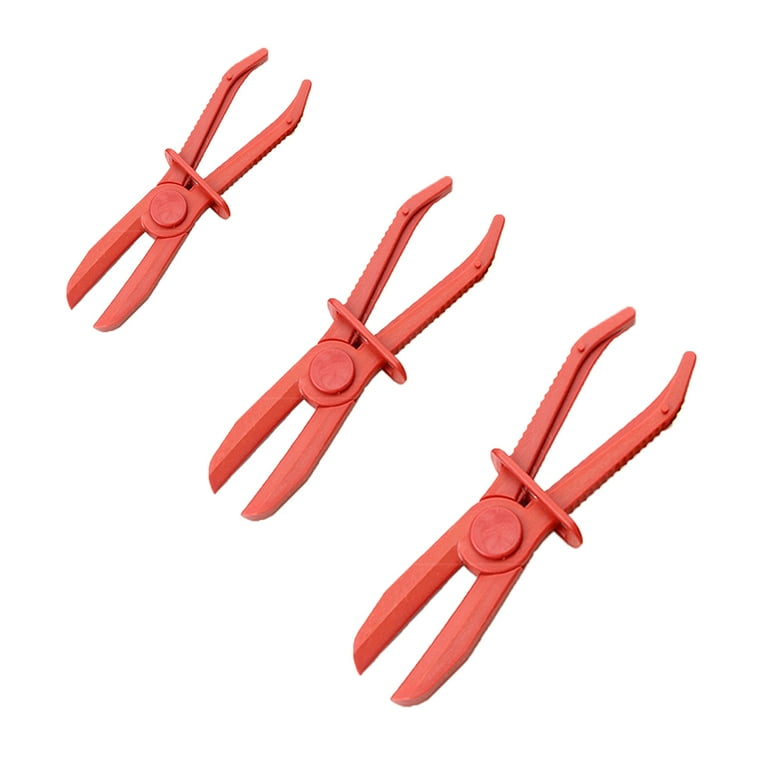This is a photo with a white background featuring three bright orange plastic tools arranged diagonally from the top left to the bottom right, decreasing in size from large to small. The tools appear to be a type of caliper or plier, each with a joint in the middle and long, narrow gripping ends. The design includes a locking mechanism or clip on the handles, allowing the tool to be secured in a closed position. Despite their simple and uniform appearance, the exact use of these tools remains unclear, though they seem to be multifunctional, potentially useful in various applications like crafts or light building tasks. The tools, while plastic and not of high quality, look sturdy enough for their intended purposes.